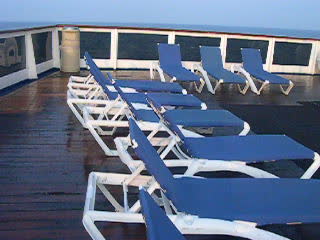The image displays a picturesque outdoor setting featuring a collection of lounge chairs arranged on a deck. These lounge chairs, often referred to as "longchairs" or "longboys," have white foundations and blue cushioned seats, adding a vibrant touch to the scene. There are approximately nine chairs in total – three facing one direction and six facing another – all placed closely together, suggesting a social or communal area. Although the image is small and the pool isn't visible, the setting strongly hints at a poolside deck or the deck of a cruise ship, especially with the blue sky and expansive water view in the background. Enhancing the idyllic atmosphere, the deck has a partition with glass panels, allowing an unobstructed view of the water, whether it’s an ocean or a lake. The wet, horizontal wooden floor further suggests recent activity or a refreshing ambience in this serene location.